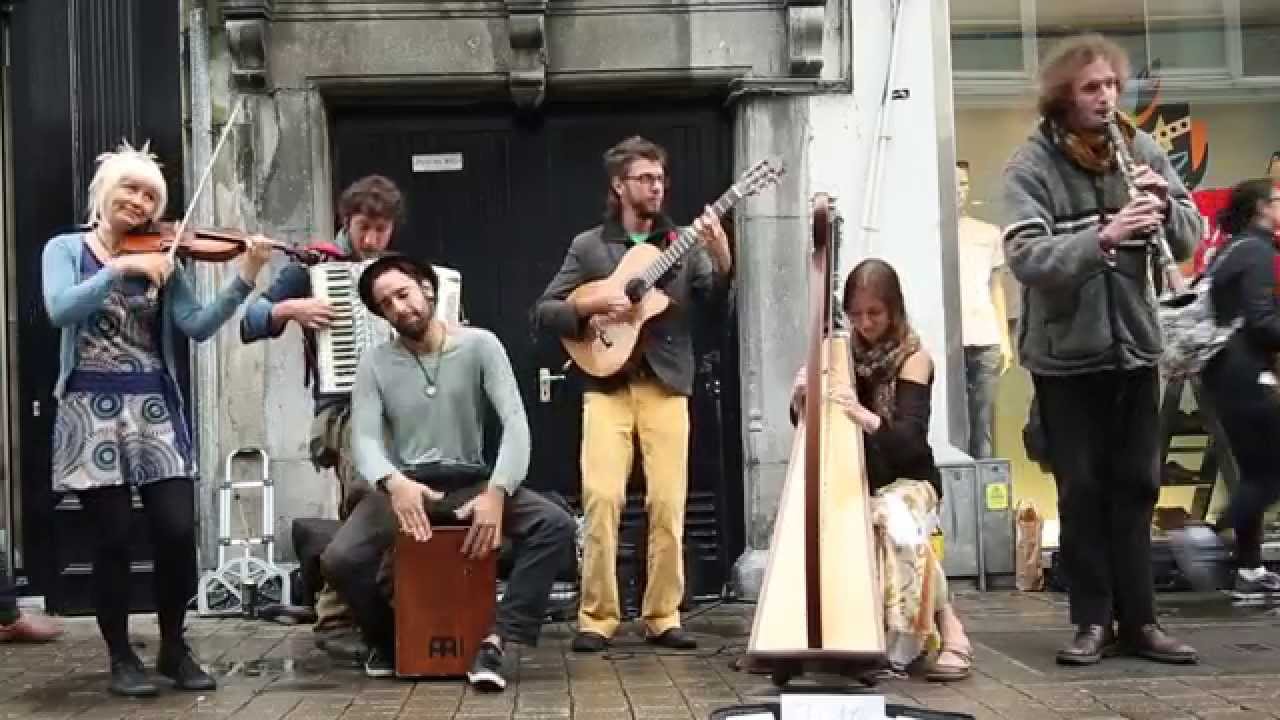This captivating photograph features a lively group of street performers possibly in a subway setting or ground level area with square stone tiles beneath their feet. In front of a backdrop of black double doors with a concrete frame, these musicians bring vibrant energy to the scene. To the left stands an elderly woman with spiked blonde hair, wearing a blue cardigan over a patterned dress adorned with blue and white circles, along with black tights and gray shoes. She passionately plays the violin. 

To her right, a man sits on a wooden block, fervently banging on it like a drum. He sports a black hat, a gray long-sleeved shirt, a necklace, dark gray pants, and black shoes, embodying a modern hipster aesthetic. Behind him, another man skillfully plays an accordion.

Further right, a gentleman in yellow Chino pants, brown shoes, and glasses strums an acoustic guitar. Among the ensemble, a woman is seated with a triangular stringed instrument, possibly a harp, while another musician, possibly playing a clarinet or trumpet, stands nearby, dressed in a gray zip-up jacket and black pants with wild hair.

The ambient environment hints at a shopping center or storefront display, with a glimpse of a mannequin in a glass window to the far right, anchoring the vibrant scene in a convincing urban landscape.